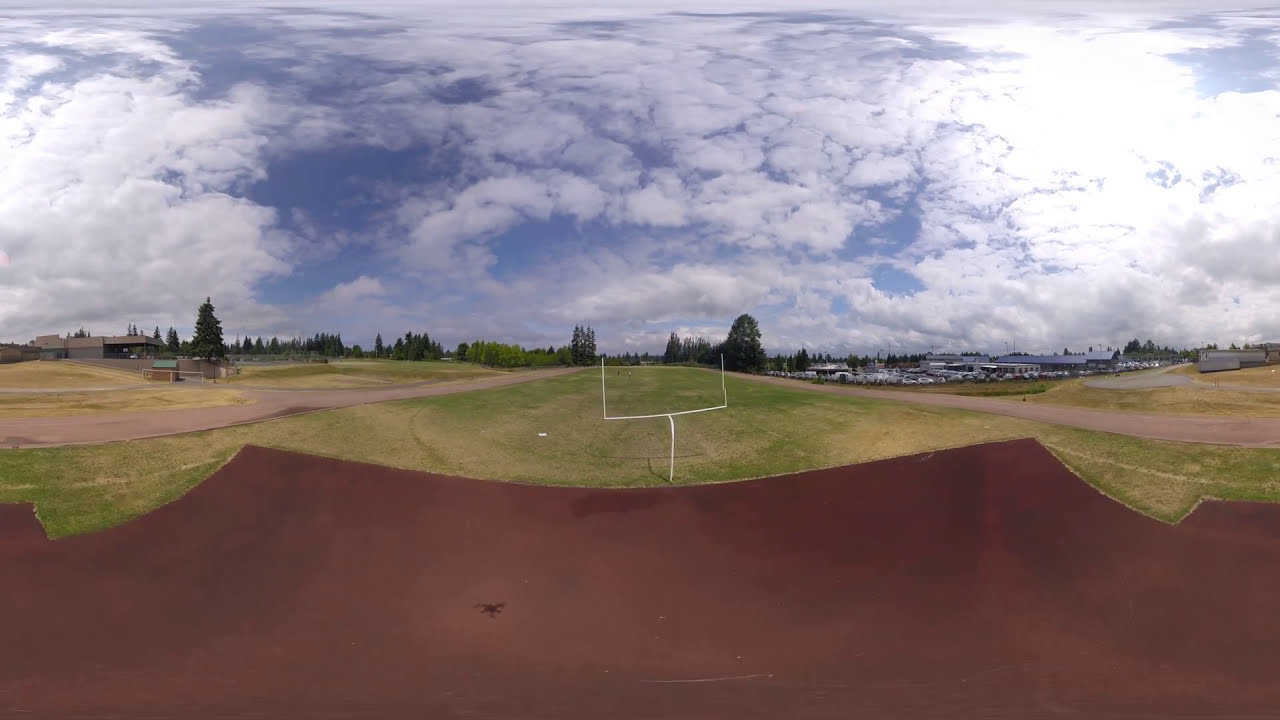The image showcases a panoramic, slightly distorted view of a football practice field taken with a fisheye or 360-degree camera, possibly by a drone. In the foreground, the ground is predominantly brown or clay-colored, resembling dirt or an uncovered area rather than traditional grass. The football goalposts are prominently visible, with one appearing curved due to the lens distortion. The field lacks typical markings or painted lines. In the background, several buildings are visible on both the left and right sides, with numerous vehicles parked, suggesting nearby parking lots or a vehicle dealership. The sky overhead is filled with clouds, allowing only patches of blue to peek through, creating a predominantly white and gray atmosphere. Additionally, roadways are seen flanking the field on both sides in the distance.